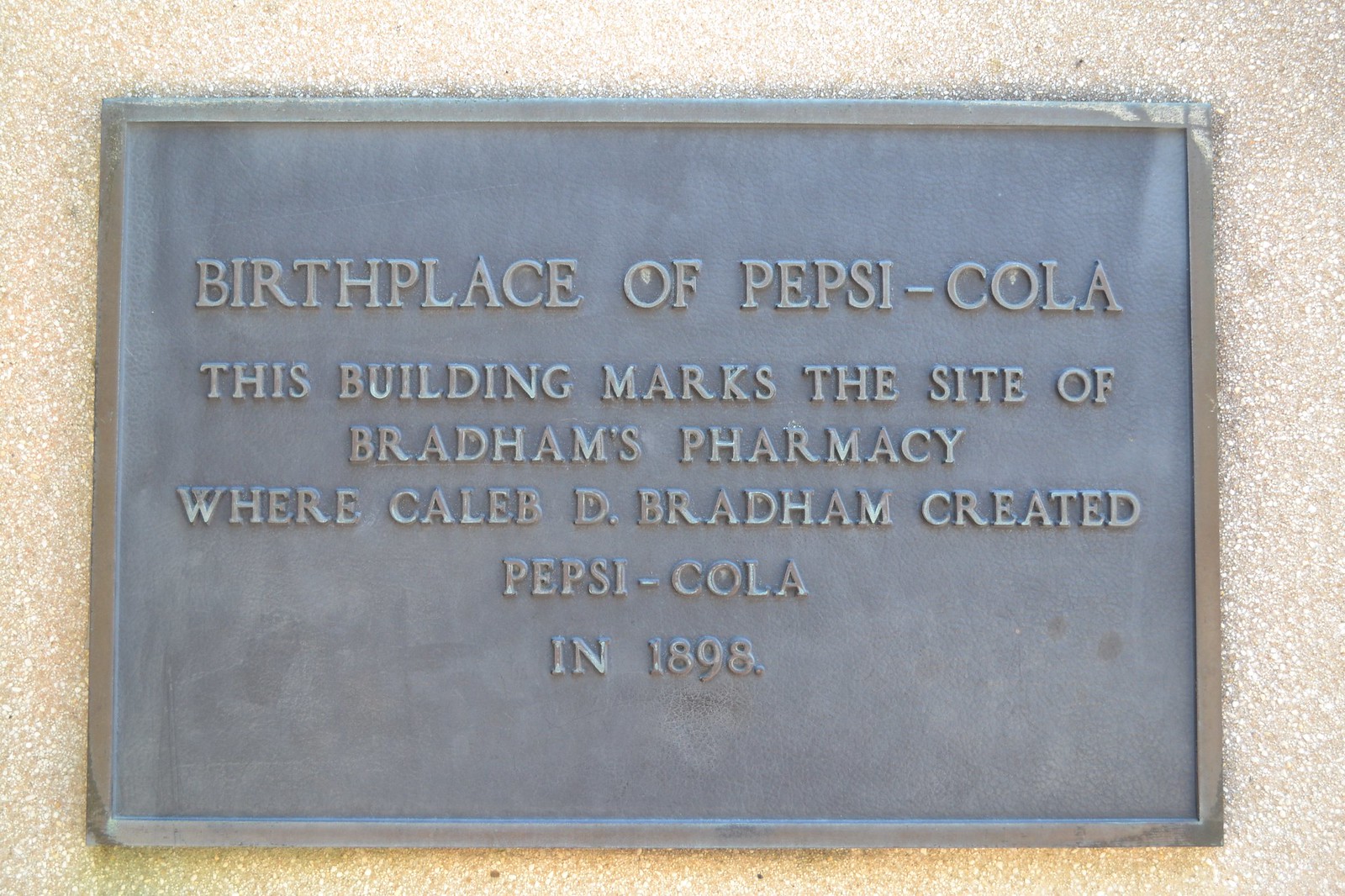This image showcases a historical plaque that commemorates the birthplace of Pepsi-Cola. The gray plaque, subtly marbled with hints of blue-gray and light blue mottling, is mounted on a concrete wall speckled with white, cream, and gray flecks. The text on the plaque reads, "Birthplace of Pepsi-Cola. This building marks the site of Bradham's Pharmacy where Caleb D. Bradham created Pepsi-Cola in 1898." The rectangular plaque features a noticeable border in the same hue, slightly textured around the text, and made of what appears to be weathered metal, possibly iron or bronze. The concrete wall behind adds a grainy and slightly pink backdrop to the scene.